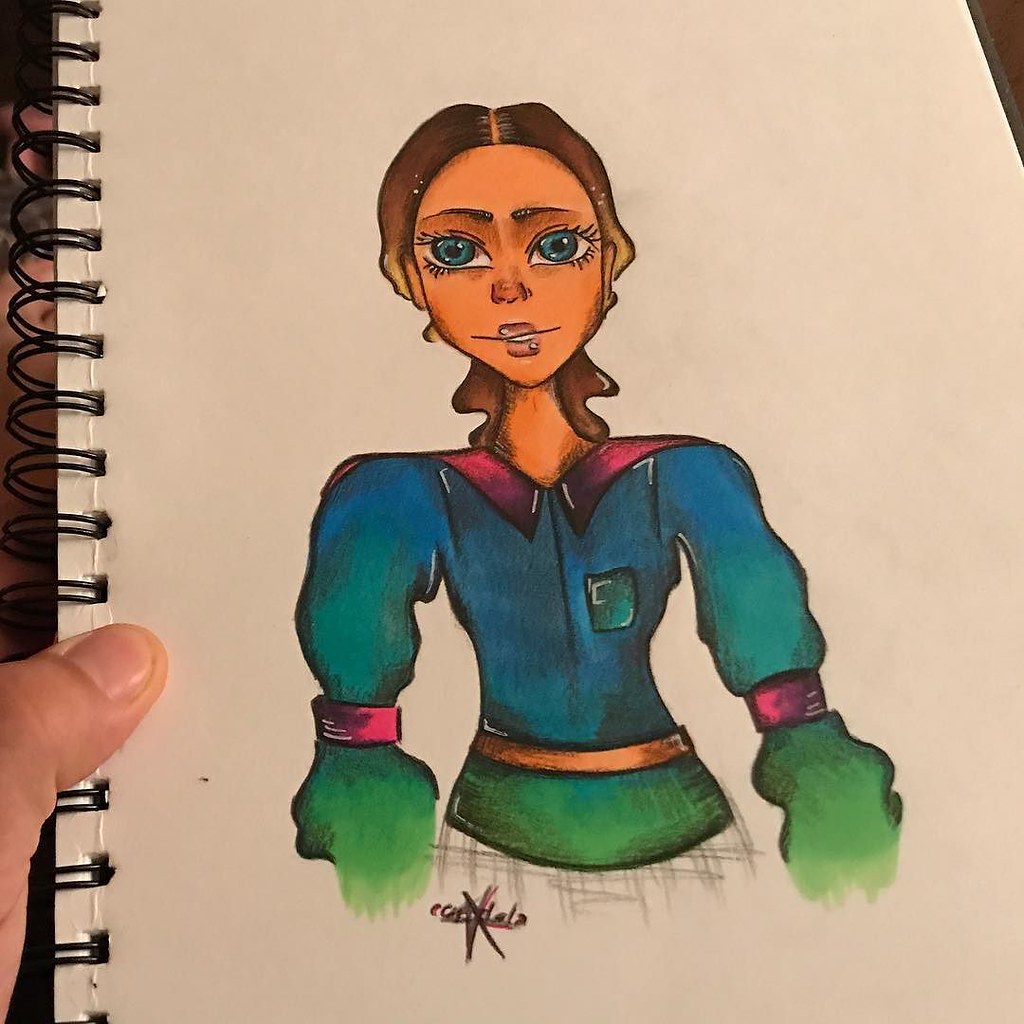This photograph captures a vibrant, hand-drawn, cartoon-style illustration created in a spiral-bound notebook. The image prominently features a colorful drawing of a woman with brown hair and strikingly large blue eyes. The artist's hand is visible on the left side of the frame, with a thumb gently holding the notebook open. The woman is depicted wearing an eye-catching shirt with a gradient effect, transitioning from blue at the top to green down her torso and arms. The shirt is adorned with additional colorful accents, including pink stripes or cuffs around the elbows and a pink collar, adding an extra layer of detail to the already vivid artwork.